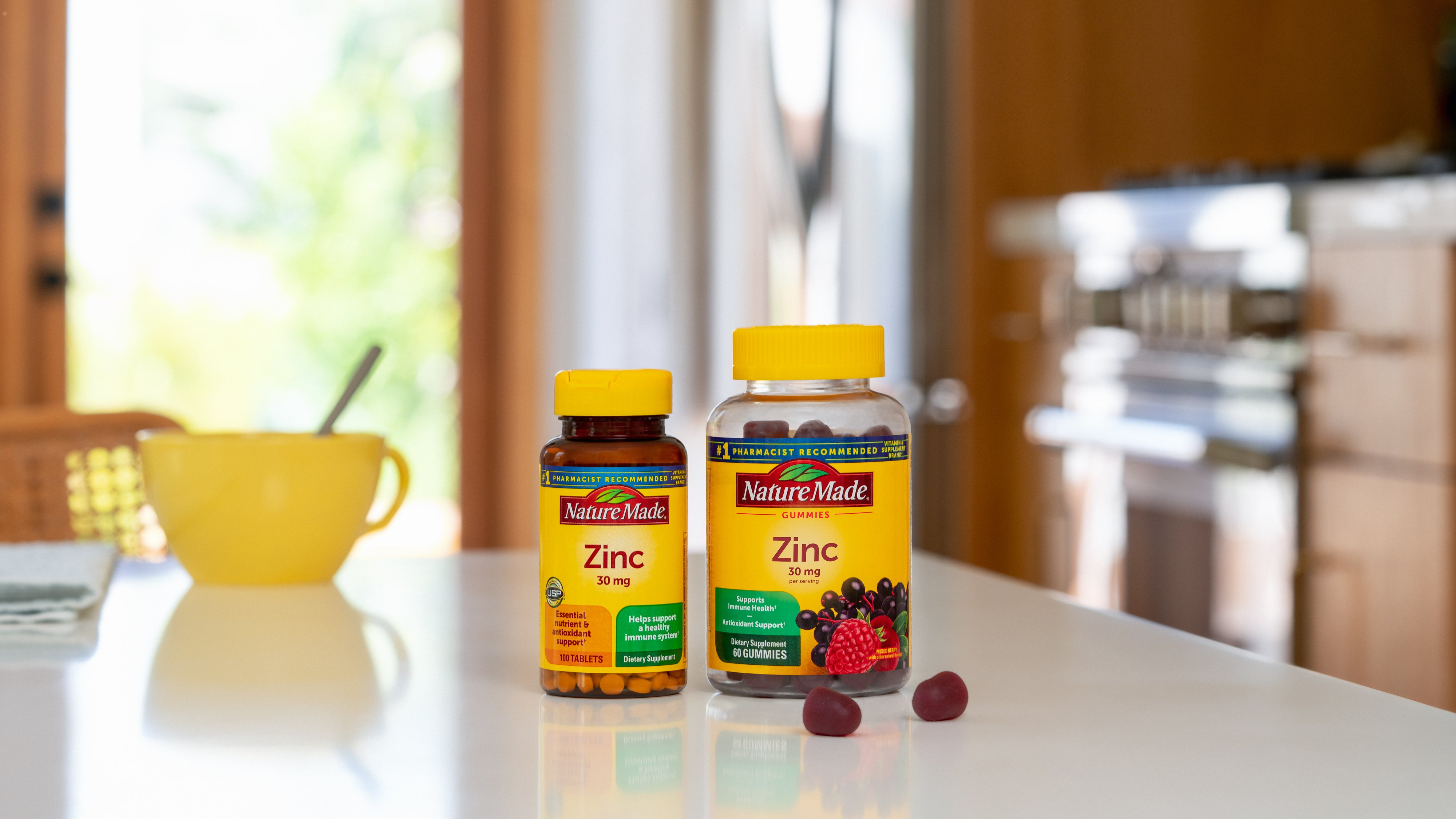This daytime kitchen scene features a pristine white countertop reflecting sunlight streaming in through a brown wooden back door on the right. Centered on the countertop are two bottles of Nature Made zinc supplements. The bottle on the left contains 100 tablets of Zinc, 30 mg, housed in a brown bottle, while the one on the right contains 60 elderberry and strawberry flavored gummies of the same dosage, in a clear bottle showcasing the red gummies. Both bottles sport a yellow label with a red rectangle at the top, highlighting the brand name and a blue banner proclaiming "Number One Pharmacist Recommended." 

To the left of these supplements, a large yellow coffee cup with a spoon sticking out is prominent, casting a subtle reflection on the glossy surface. In the background, a stove and additional wooden cabinets can be seen, along with a rustic style seating area draped with a folded cloth napkin. Two red gummies lie on the countertop just in front of the gummy bottle, emphasizing the product's form and flavor. The natural light flooding through the door amplifies the clean and bright ambiance of this homey kitchen setting.